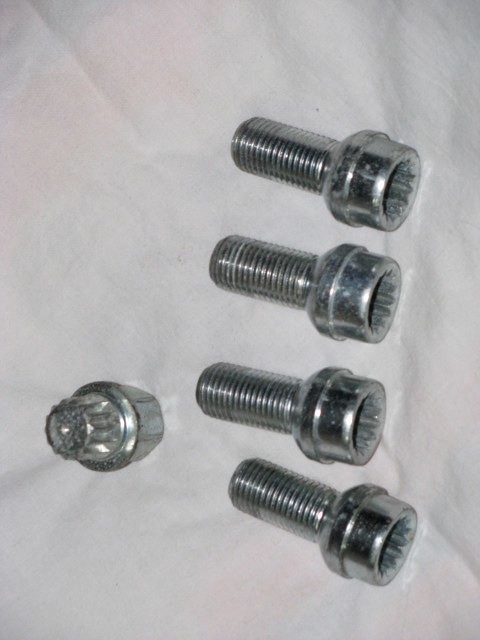The image displays five silvery metallic screws arranged on a white backdrop that has a subtle light pinkish tinge, resembling a piece of cloth or material like a pillowcase or sheet. Four of the screws are lined up vertically, one beneath the other, and all are oriented in the same direction. The fifth screw stands out, positioned upright on its bottom. The screws have cylindrical bodies with threaded surfaces and rounded tops with central holes. Additionally, to the left of the screws, there's an object resembling a vintage faucet handle with a cut-glass design, suggesting the screws might be related to bathroom fixtures. The image is zoomed in, making the screws appear larger than their actual size.